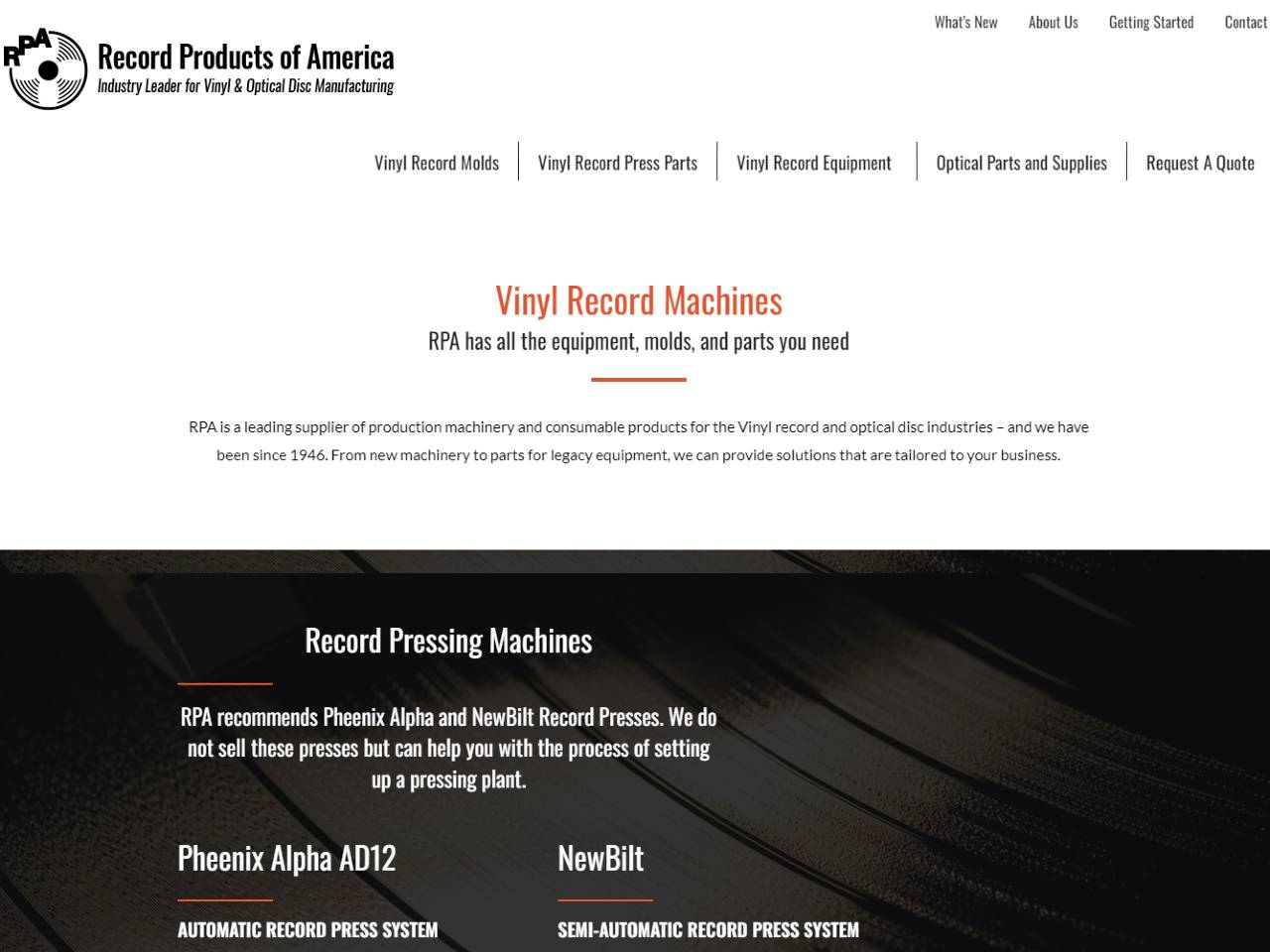**Descriptive Caption:**

This image is a screenshot of a detailed webpage for "RPA - Record Products of America," highlighting their expertise as an industry leader in vinyl and optical disc manufacturing. On the left side, there is a prominent image of a vinyl record with the text "RPA" and "Record Products of America - Industry Leader for Vinyl and Optical Disc Manufacturing" in bold black letters. 

To the right, in small gray letters, the website menu lists options such as "What's New," "About Us," "Getting Started," and "Contact." Directly beneath these options, tabs are displayed offering links to various sections: "Vinyl Record Molds," "Vinyl Record Press Parts," "Vinyl Record Equipment," "Optical Parts and Supplies," and "Request a Quote."

Highlighted in bold orange letters is the heading "Vinyl Record Machines," accompanied by the statement: "RPA has all the equipment, molds, and parts you need." Below this heading, a detailed description reads: "RPA is a leading supplier of production machinery and consumable products for the vinyl record and optical disc industries and we have been since 1946. From new machinery to parts for legacy equipment, we can provide solutions that are tailored to your business."

The background of this section features an image resembling a vinyl record, reinforcing the theme. Text within this section specifies "Record Pressing Machines" and recommends two specific models: "Phoenix Alpha AD 12" and "New Built." It clarifies, "We do not sell these presses but we can help you with the process of setting up a pressing plant." Additional information labels the Phoenix Alpha AD 12 as an "Automatic Record Press System" and the New Built as a "Semi-Automatic Record Press System," completing this in-depth overview of RPA's offerings.